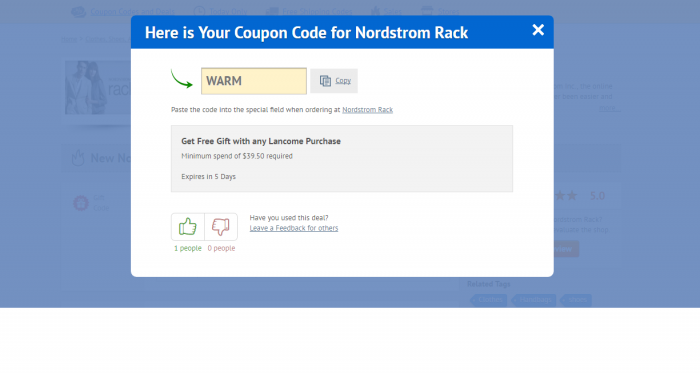The image depicts a web page displaying a promotional coupon code for Nordstrom Rack. The background of the page features a muted blue tone with a partially visible image of a man and a woman standing beside each other. The word "NEW" appears prominently, alongside an illustration resembling flames and a 5.0-star rating.

At the forefront, there is a white pop-up box. The top section of this box has a blue banner with white text that reads, "Here is your coupon code for Nordstrom Rack." The coupon code, "WARM," is highlighted in a yellow rectangle. A green, curved arrow points downward toward the coupon code.

Below the coupon code, there is a button labeled "Copy," followed by the instruction: "Paste the code into the special field when ordering at Nordstrom Rack." Additionally, it mentions an offer: "Get a free gift with any Lekoma purchase."

At the bottom of the pop-up, there are two buttons for user feedback: a green thumbs-up for approval and a red thumbs-down for disapproval.